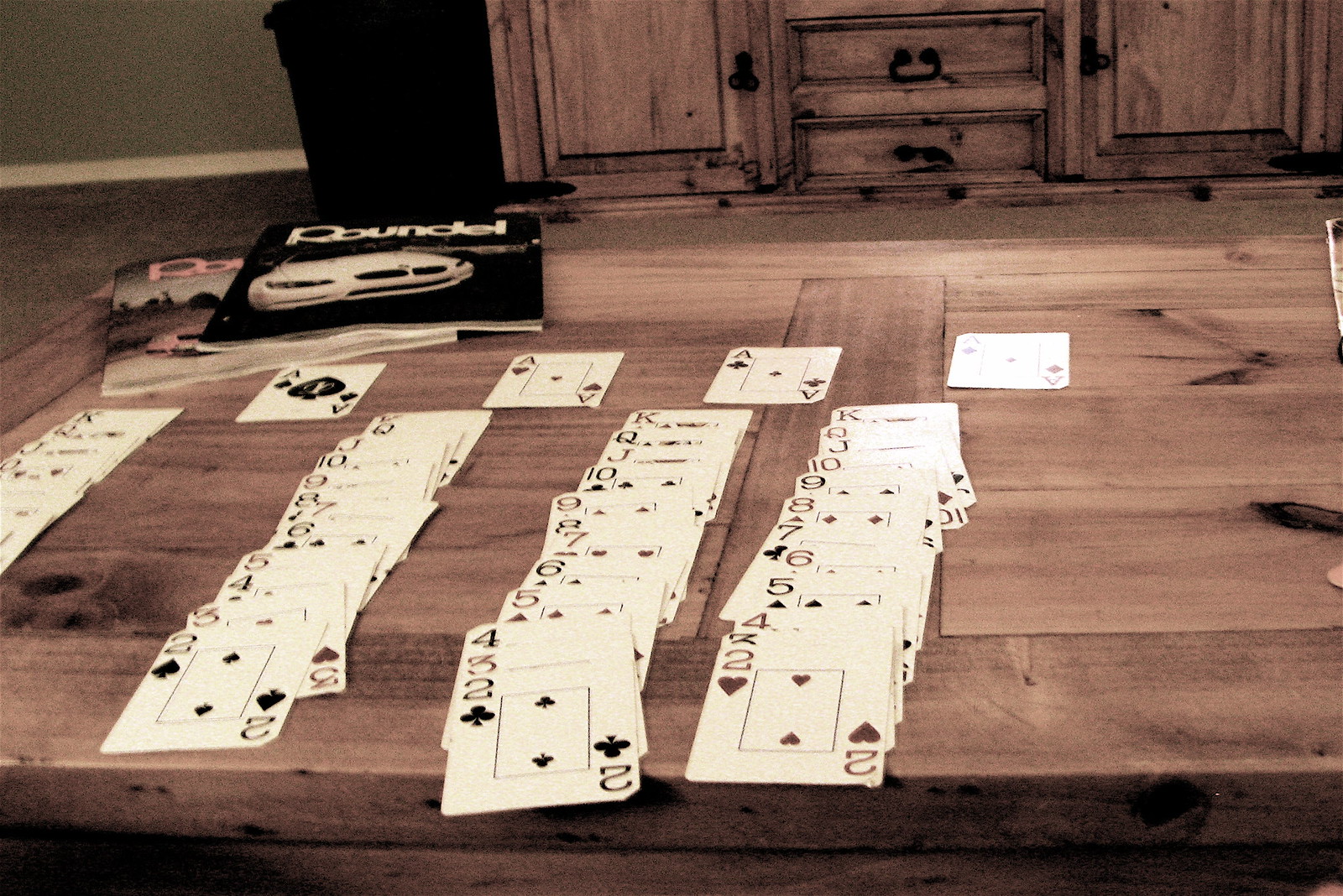The rectangular image captures a victorious game of solitaire displayed on a wide wooden coffee table. The long side of the rectangle stretches horizontally. All four suits are meticulously arranged, featuring alternating colors from Kings down to Twos, signifying that the game has been won. Above these organized rows of cards are the four Aces, marking the columns' start. The Twos visible include the Two of Hearts, Two of Clubs, and Two of Spades, with the partially seen Two on the far left.

In the left-hand corner of the table, two magazines lie stacked with a few cards resting on top of them. The table is set against a background showcasing a brown carpeted floor and a light green wall adorned with white trim at the base. A cabinet, possibly for a TV, stands against this wall, equipped with several drawers and cabinets. At the left side of this cabinet, a black box can be seen.